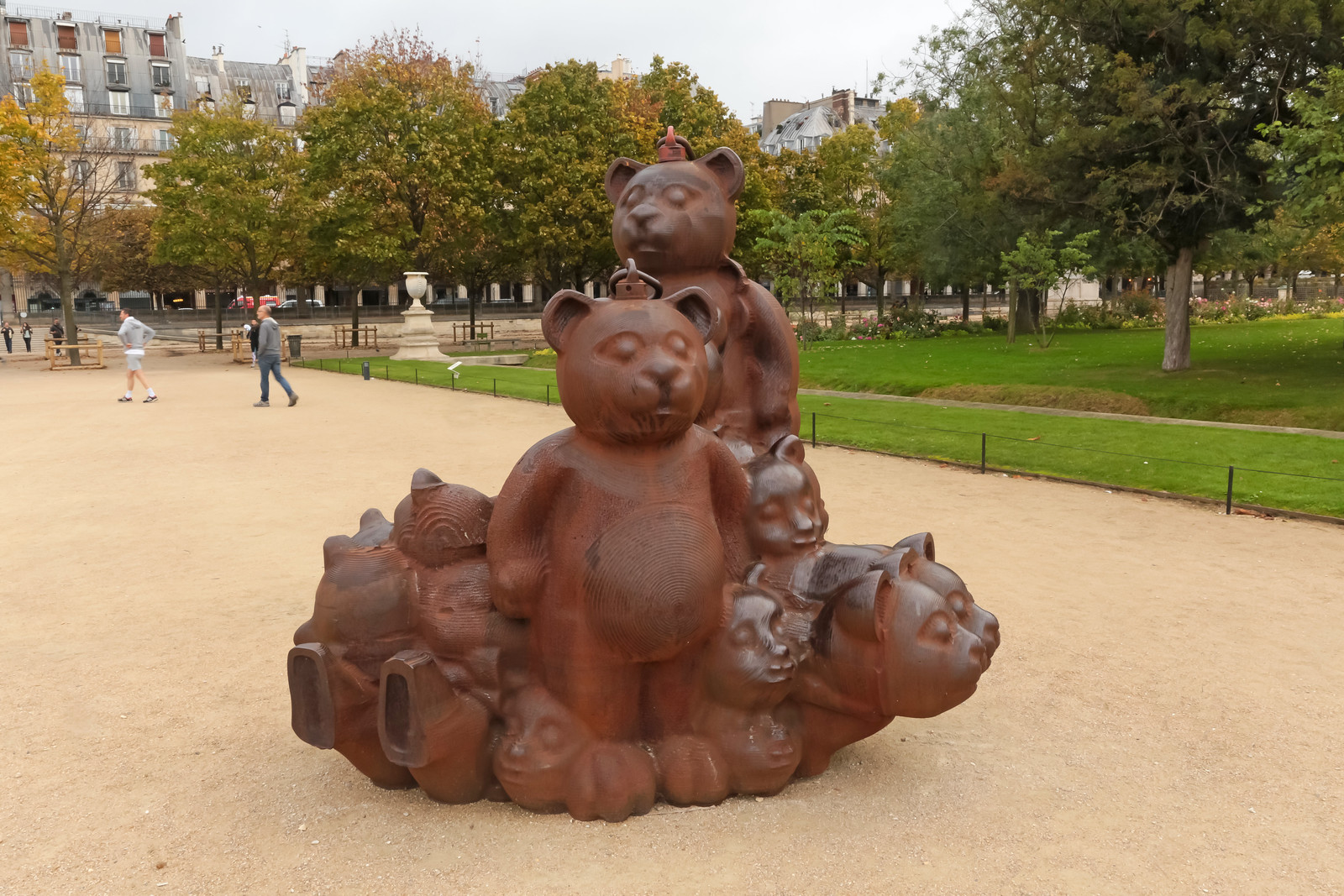In this slightly sunny, AI-generated photorealistic image, we see an outdoor park showcasing a unique statue of humanoid bear figures. The scene features a mix of green and autumnal orange trees partially obscuring some inconsistently shaped buildings in the background. The park itself has healthy green grass and a sandy dirt path in the foreground, where two individuals, one dressed in a suit and the other in shorts and tennis shoes, are walking. At the center of the image is a modern, unsettling sculpture made of rusted iron or terracotta, displaying a group of bears. Two large bears stand prominently, with numerous bear heads clustered around their lower bodies, creating a layered and chaotic effect. The sky above is white, adding to the eerie, surreal atmosphere of the scene.